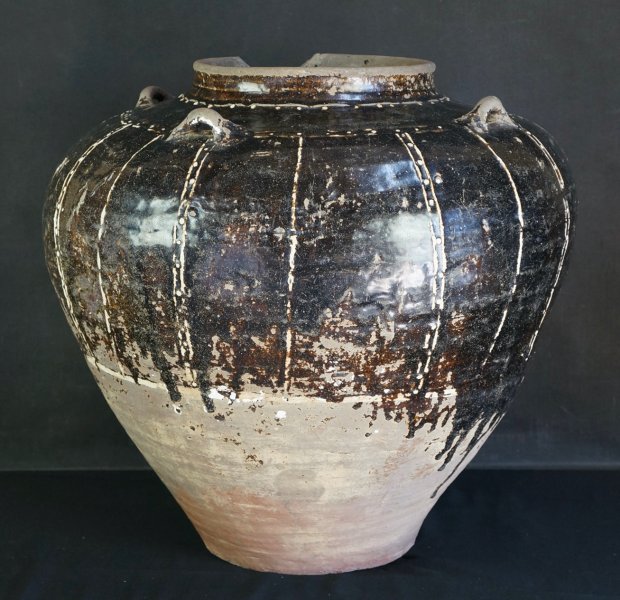The image features a large, ancient vase with a distinctive shape, broader at the top and tapering to a smaller base. The vase has a worn appearance, particularly at the bottom, where the original paint has faded, revealing a beige, weathered surface. The top part of the vase exhibits a dark brownish-black color, heavily weathered with splotches. White vertical stripes descend from the top towards the middle, breaking through the dark upper section. There is a noticeable chip on the vase, adding to its aged appearance. The vase features an open, rimmed lip at the top and has three small handles or hanging notches, likely used for placing string or hooks for display purposes. The background is entirely black, with a dark gray wall and a black floor, emphasizing the solitary presence of the vase with no other objects in the frame. The glossy sheen on the vase suggests it may have been glazed at some point, although this has also worn with time.